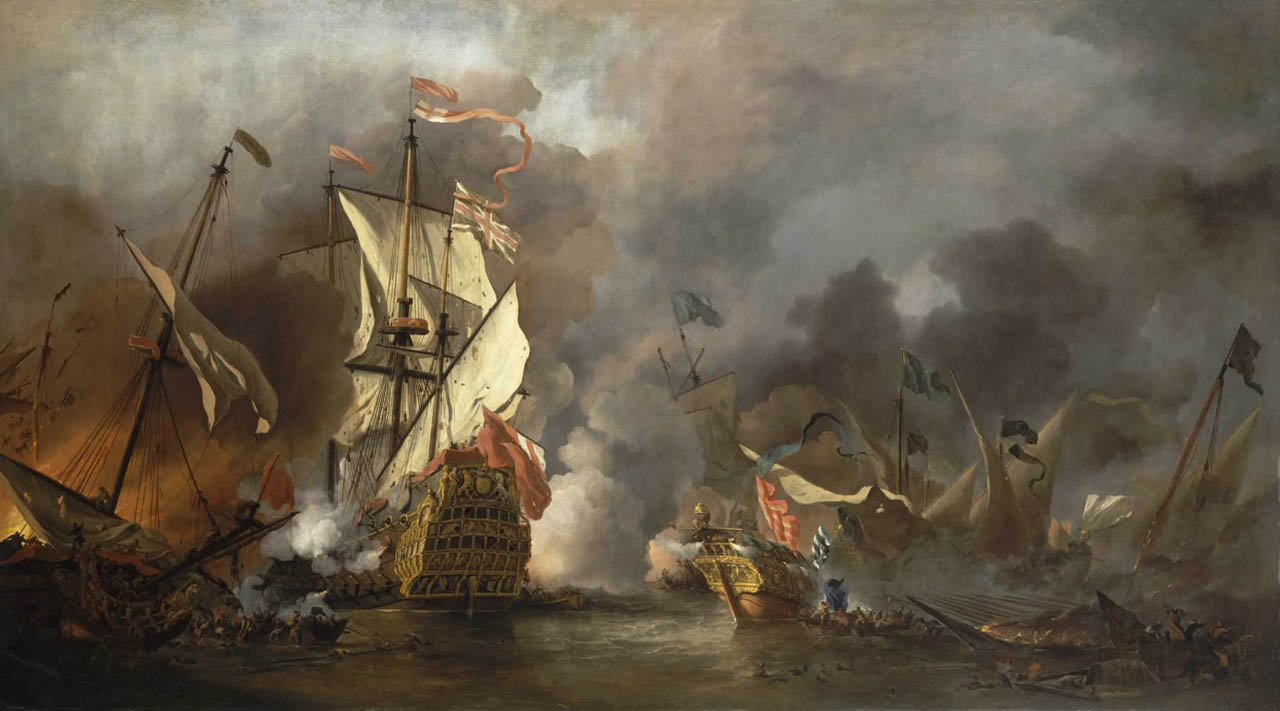The image captures a dramatic scene from an old rectangular painting measuring approximately six inches wide by three to four inches high. It portrays a fierce naval battle against a backdrop of a gloomy, cloud-covered sky filled with thick smoke. The lower half-inch of the painting features dark gray waters. On the left side, a sailing ship is depicted in the process of sinking, with its torn sails barely above the water and people frantically jumping into a lifeboat. The center of the scene is dominated by a seemingly intact sailing ship flying the British flag. This ship is firing its guns, evidenced by white smoke billowing from its sides. To the right, more sunken ships are visible, some bearing black or blue flags, with survivors attempting to reach rowboats. The entire scene is enveloped in shades of gray, with occasional patches of white and red, particularly on the left side, further enhancing the chaotic atmosphere of the battle.